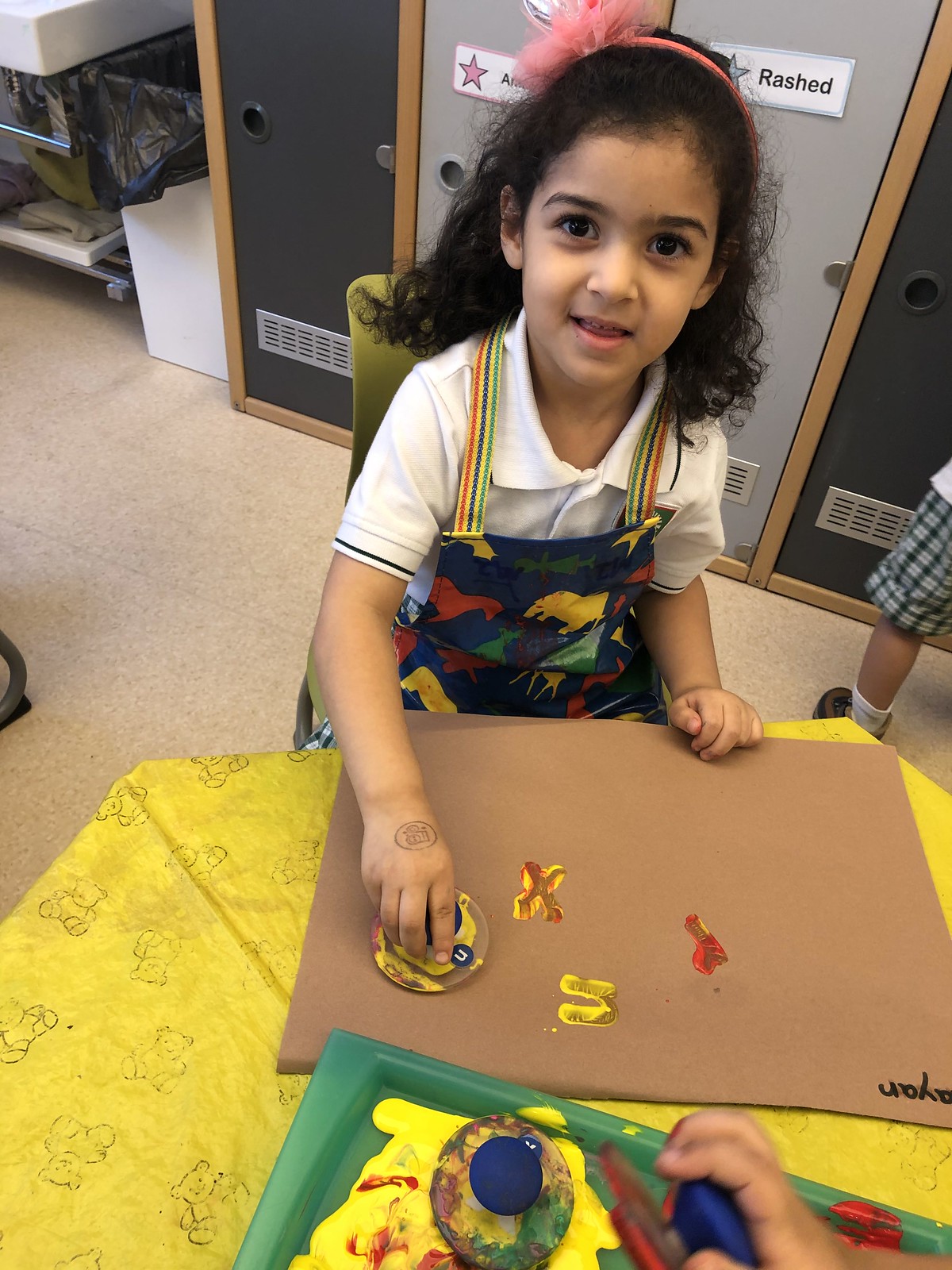In a cheerful kindergarten classroom, a young girl, likely around six or seven years old, is captured in a moment of creativity. She sits at a yellow craft table covered with a brown mat, diligently working on an art project. In front of her lies a piece of brown construction paper, which she is decorating with colorful Play-Doh and paint. Her hands, adorned with traces of paint, are busy stamping patterns onto the paper.

The girl wears a painter's overall, vibrant with smudges of red, green, and yellow from past endeavors. Beneath the overall, a white t-shirt with a collar peeks out. Her ensemble is completed with a pink frilly lace bow headband perched atop her wavy, curly brown hair. She smiles gently at the camera, exuding joy and concentration. 

In the background, beige flooring leads to a row of lockers, one notably labeled "Rashad" with a blue star. A glimpse of another child’s fingers maneuvering blue Play-Doh adds life and context to the scene, highlighting the communal and playful atmosphere of the classroom. This snapshot beautifully encapsulates the innocence and creativity of childhood.